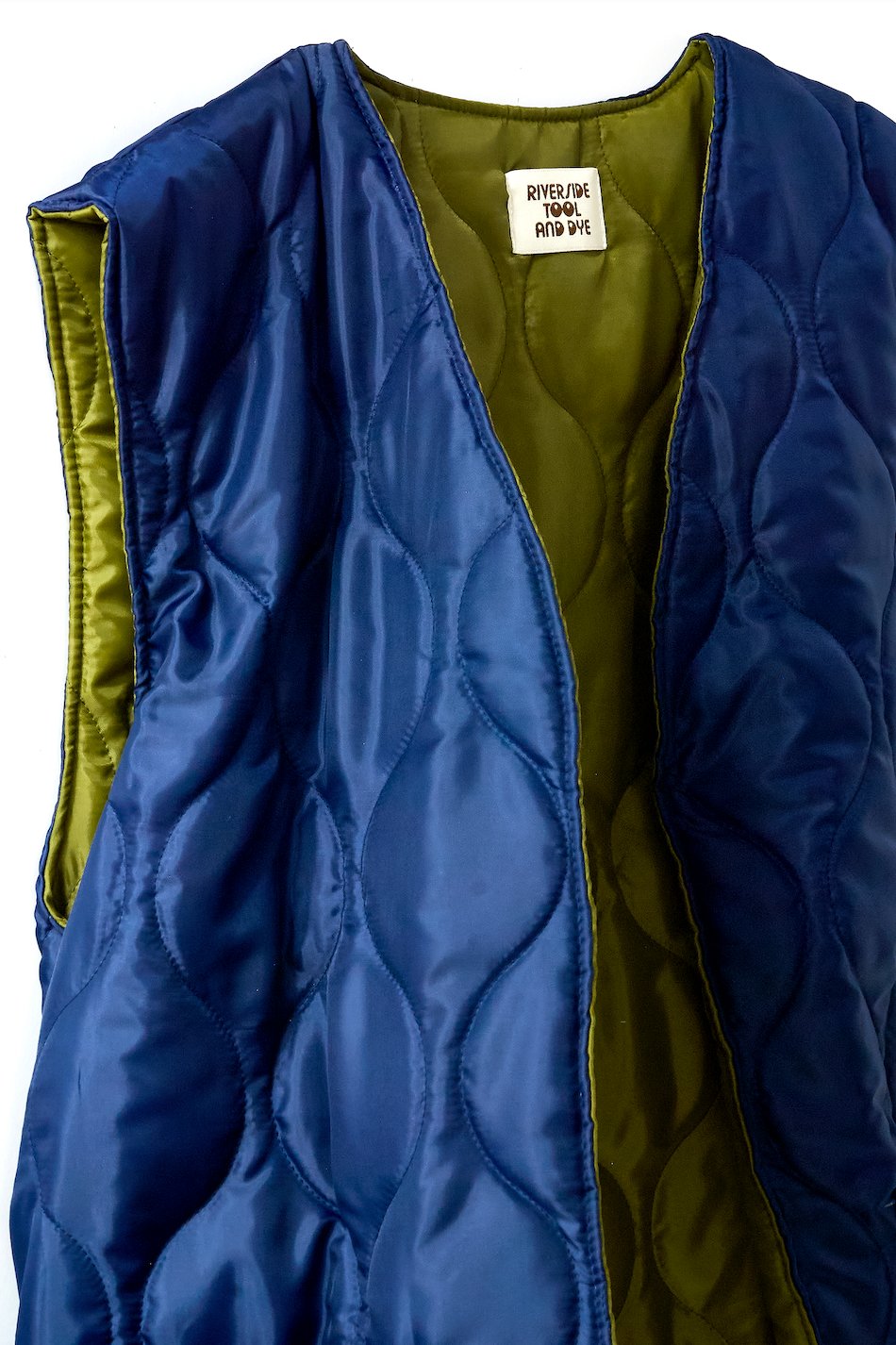The image showcases a close-up photograph of an outdoor vest, set against a solid white background that takes up most of the frame. The vest itself, likely featured for a website, is made of high-quality, insulated material characterized by a repeated hourglass stitch pattern. The exterior is a shiny blue, while the interior is a glossy olive green. A white tag located at the top of the vest bears the branding "Riverside Tool and Die." Due to the close-up nature of the photo, only the left-hand side of the vest is fully visible, and the complete view of the right side and bottom is outside the frame.